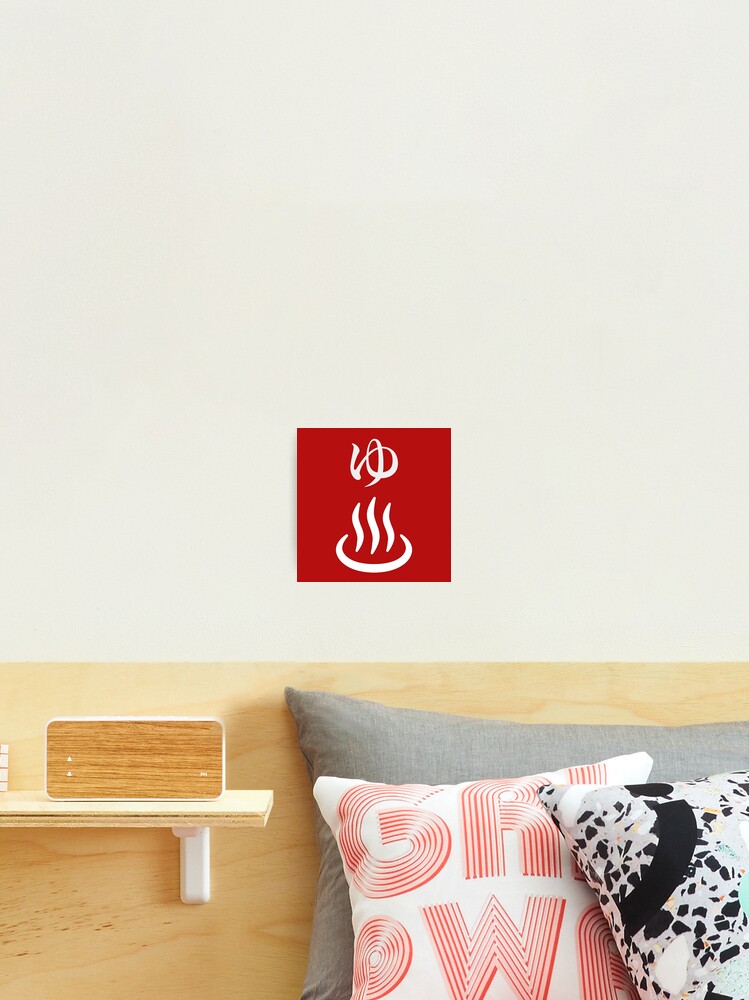The photograph captures a serene bedroom scene featuring the headboard section of a bed and the surrounding wall. The top half of the wall is painted white, contrasting with the pale wooden headboard beneath. A small, modern wooden shelf, supported by sleek brackets, is attached to the wall above the headboard. On the shelf sits a modern alarm clock with a wooden facade and white digital displays, currently not showing the time. Above the shelf, a red picture adorns the wall, showcasing two graphic images within, the details of which are difficult to discern but might resemble a cup with steam rising from it.

Resting against the solid, flat plank headboard are several pillows. A prominent larger gray pillow serves as a backdrop for two smaller ones in front. One of the smaller pillows is white and features graphic pink lettering that begins with "GRW," though the rest is illegible. The other smaller pillow is white with black designs that appear speckled, giving it a textured, modern look. The combination of the minimalist wall decor, the natural wood elements, and the eclectic pillow designs create a cozy and stylish ambiance in the room.